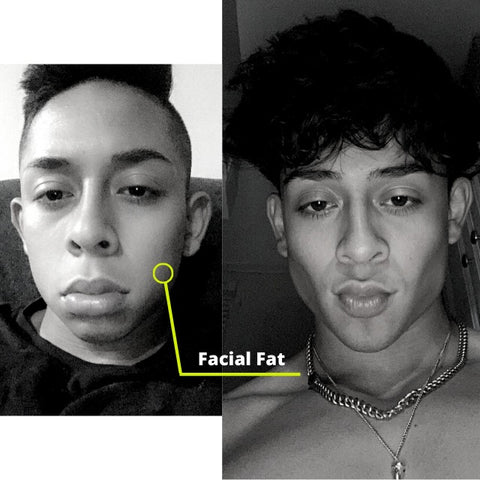The black and white photo consists of two side-by-side images of a young, Latin or Spanish-looking man, functioning as a before-and-after comparison. Both images are clear and well-lit with natural lighting. In the left image, the man's face appears fuller and rounder, with a yellow arrow pointing to his cheek labeled "facial fat." The right image shows the same man, but with a more chiseled and defined jawline, indicating a significant reduction in facial fat. The differences are also highlighted by the changes in his hair length; it is shorter in the left image and longer in the right, making him appear slightly older.